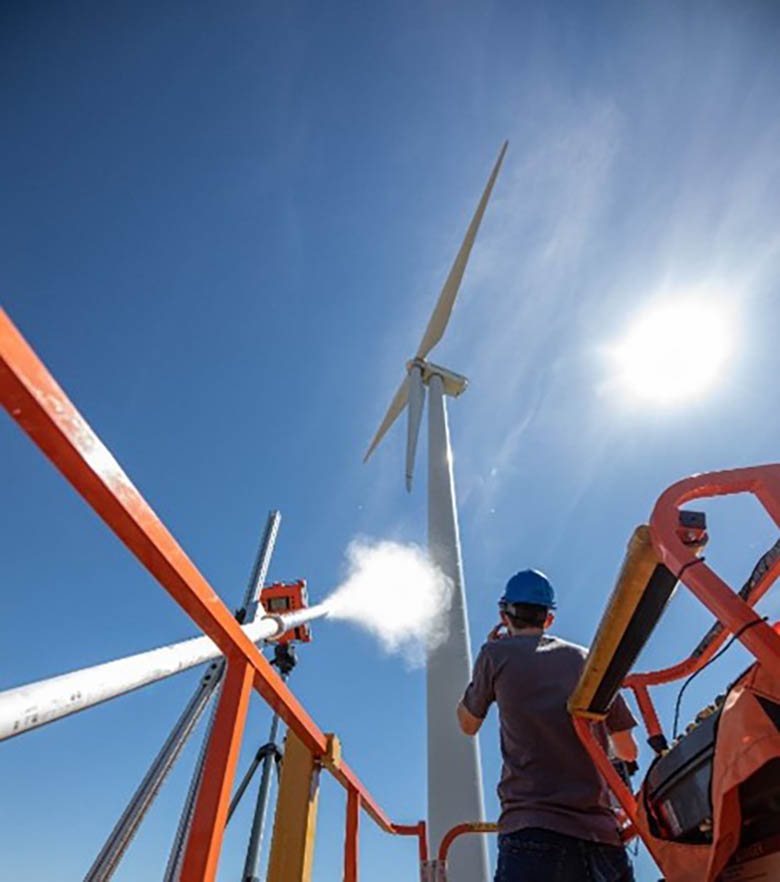In this vertical rectangular image, we see a construction worker standing on an orange-framed lift with a railing, working on the installation of a wind turbine. The silver base of the turbine stretches upward, with three blades already attached, indicating the ongoing process of blade installation. The worker, dressed in a gray t-shirt, gray pants, and a blue hard hat, stands with his back to us, gazing up at the turbine. The lift he is on includes a cabin where the controls are located and features an orange railing around it. To the left of the image, a white hose is present, emitting steam or gas that rises toward the top right. Additionally, there's a section of railing which is yellow, and a mechanical lift device with tripod legs can be seen in the background, suggesting it assists workers in reaching the turbine's height. On the right side of the image is a machinery piece with an orange frame and a black section with buttons, likely part of the construction equipment. The sky is visible in the background, casting natural light over the scene.